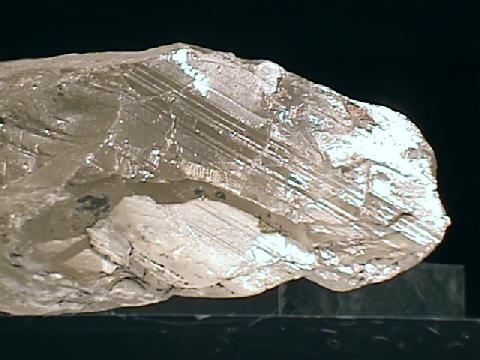The image depicts a long, flat rock or potentially an unrefined gem, with distinctively diagonal striations and a surface that appears unpolished. The rock starts on the left and extends towards the right, where it becomes more rounded and oval-shaped. The upper left section of the rock is brownish-gray, transitioning to a very bright, iridescent white at the upper right tip. The rock is set against a black background, and it appears to be placed on a dark, possibly marbled surface. The entire rock isn't visible, as it seems cut off at the left edge, suggesting it might be a precious or semi-precious sample displayed for viewing.